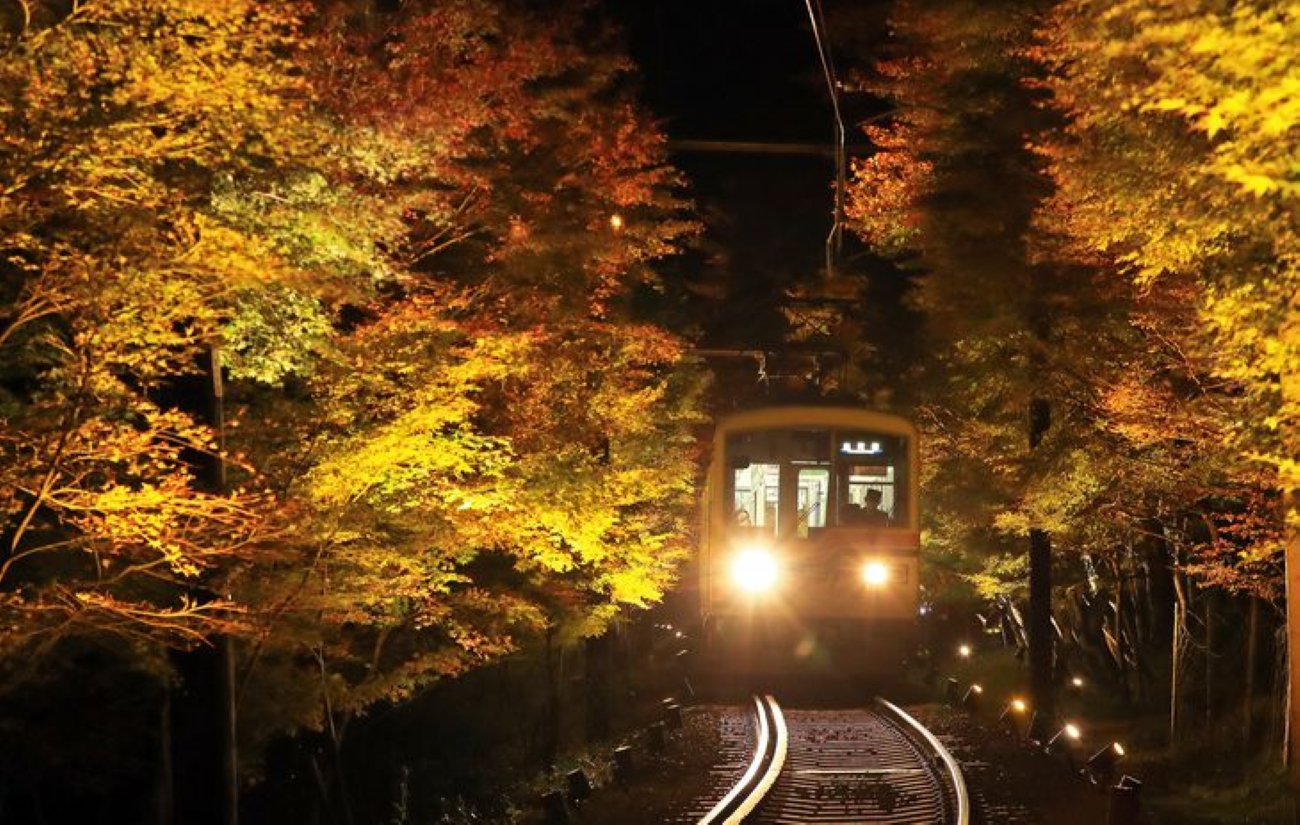An electric train with a bright yellow front and two illuminated headlights drives through a forest at night. The box-shaped rail car, resembling a subway car, has an arm connecting to an overhead wire. Inside, the silhouette of the conductor can be seen, possibly wearing a hat, and there might be a few passengers visible. The tracks curve toward the train, leading it through a tunnel of vibrant autumn trees with leaves in shades of yellow, orange, and red. The dark sky above and the shadows cast around the trees highlight the contrast of the train's bright lights cutting through the night. In the background, some distant lights can be seen, further emphasizing the isolation of the scene.